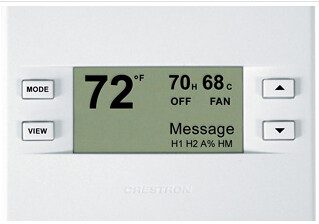This is a detailed photograph of a digital thermostat, set against a pristine white background, likely for an advertisement. The thermostat features a sleek design with several controls and a digital display at its center. On the far left are two buttons labeled "Mode" and "View". On the far right, there are two buttons marked with an up arrow and a down arrow, presumably for adjusting the temperature settings. The central digital readout window indicates the current room temperature as 72 degrees Fahrenheit, with the thermostat itself set to 70 degrees Fahrenheit, though the heating system is currently off. Additionally, the fan is set to 68 degrees Fahrenheit. The display also shows various status messages including "H1," "H2," "8%," and "HM." The thermostat is predominantly white, with a subtle brand name inscribed in gray at the bottom, which appears to begin with the letter "G" but is faint and somewhat difficult to discern.